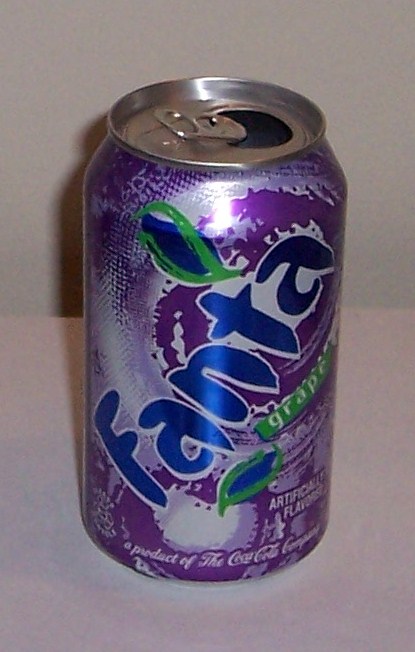The image features a vibrant purple Fanta can adorned with intricate purple swirls. The iconic Fanta logo, set with bold blue letters outlined in white, slants diagonally from the bottom left to the top right of the can. Flanking the logo are stylized, leaf-like shapes in blue, bordered by a green outline. Just below the final letters of the Fanta logo, the word "Grape" is prominently displayed in white text, set against a green stripe backdrop. The can has been opened, and near its bottom, there is a clear message stating, "A product of the Coca-Cola Company," with a note about "Artificial Flavors" positioned slightly above it. The entire can exudes a lively, eye-catching design synonymous with the Fanta brand.